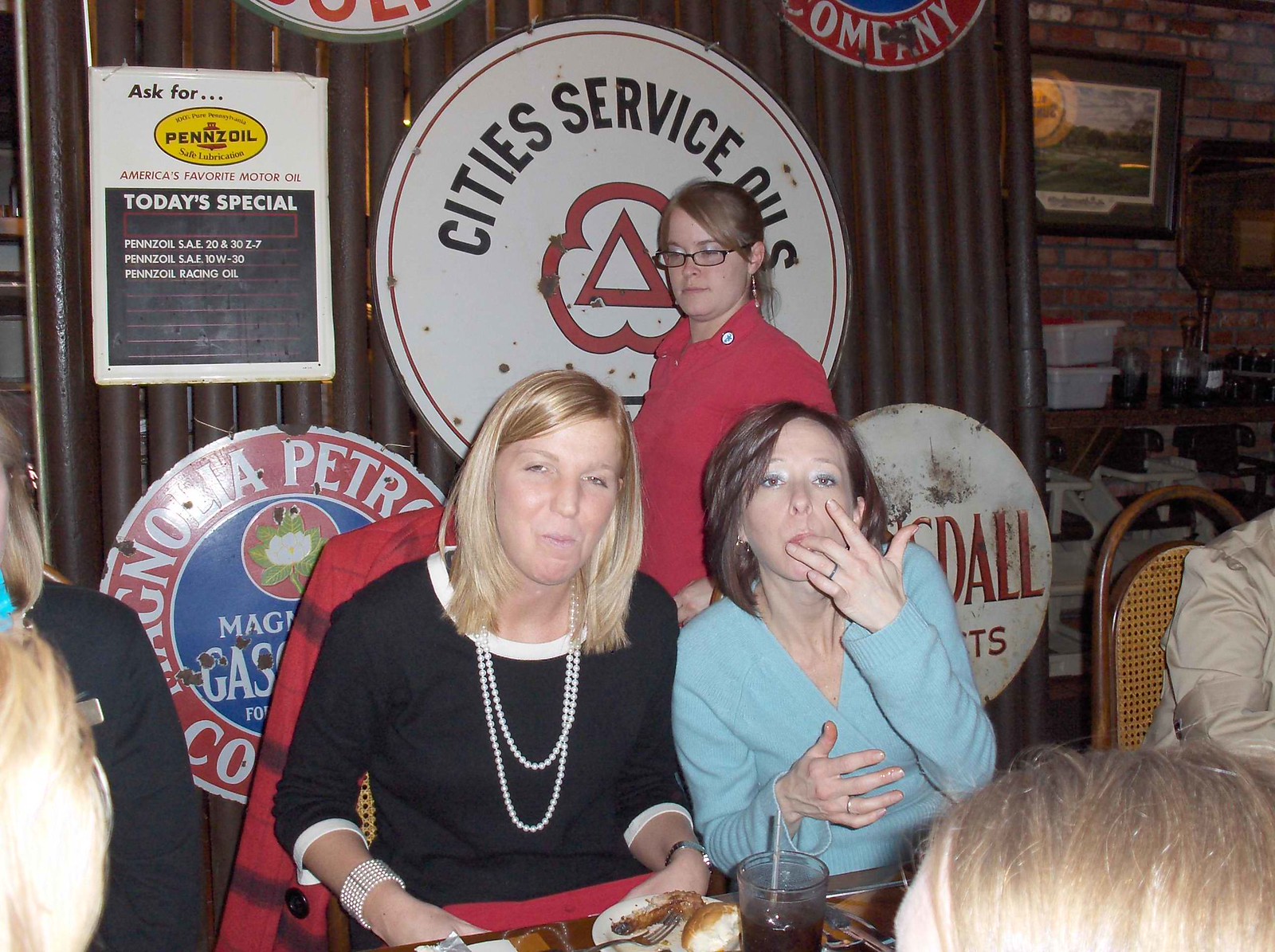This horizontal-rectangular photograph captures a busy scene inside a restaurant. In the forefront, two women are seated at a table, engaged in their meal. The woman on the left has long blonde hair, is wearing a black top adorned with two strings of pearls, and her hands are occupied as she appears to have her mouth full. Beside her, the woman in the blue top, who has darker hair, is seen licking her fingers, suggesting she just placed something in her mouth. The table in front of them displays various food and drink items.

Standing behind these two women is another person who might be a server, though their gender is ambiguous. The background is bustling with the heads and partial views of other patrons. The wall behind them is decorated with several circular signs and posters. Prominently, a large white circular sign in the center reads "City Services." Other circular signs are visible, including one with red text on the left and another with white text on the right. A prominent red triangle with a three-leaf clover shape surrounds it. To the left, a blackboard-like sign announces "Today's Special," beneath another poster promoting Penzoil, America’s favorite motor oil, including its price.

This lively image captures a candid moment in a restaurant filled with vibrant wall decor and the dynamic interaction of its patrons.